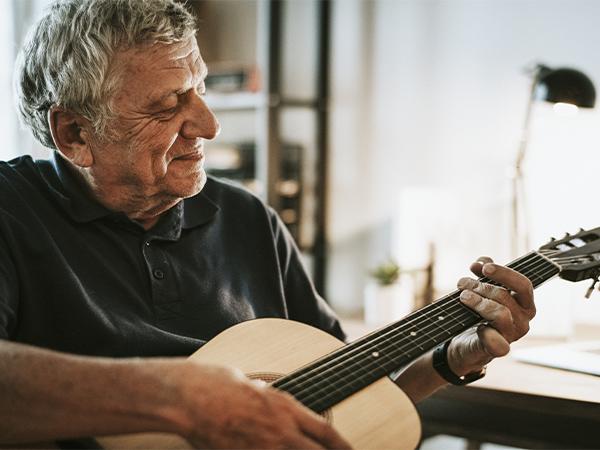The image captures an elderly man deeply engaged in playing his guitar, exuding a serene and focused demeanor. Wearing a black polo shirt, he showcases his salt-and-pepper, wavy gray hair, along with distinguished features such as bushy eyebrows, a long drooping nose, and deep wrinkles around his eyes and forehead. Seated in an office chair, the man holds a brown and black guitar in both hands, his left hand working the frets while his right hand strums the instrument. His gaze is fixed downwards at his left hand, and there's a hint of a smile on his face. In the background, a small office table is visible, adorned with a long-necked lamp with a black shade, a set of shelves, a cabinet door, and a small plant. The man also sports a black watch on his left wrist.